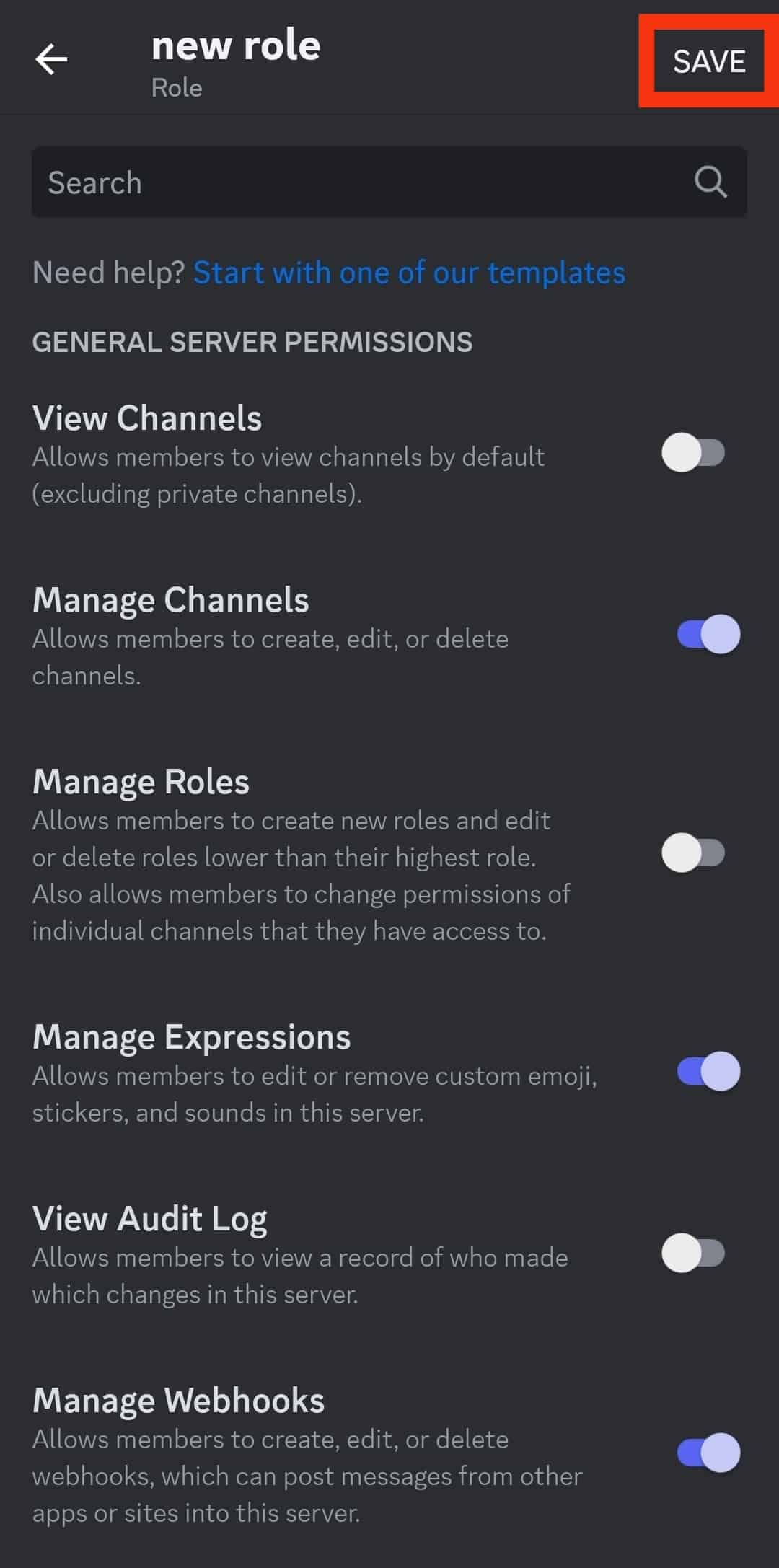The image showcases a settings screen on a phone with a dark gray background. At the top, there is a white arrow pointing left, followed by the text "New Role" in white and "Role" in gray beneath it. On the far right, the word "Save" appears, highlighted by a red marker box.

Below this, a black banner includes the word "Search" in gray with a search icon on the right side. Further down, the background returns to dark gray, displaying the text "Need Help" in light gray, followed by a blue link that says, "Start with one of our templates."

Continuing downward, "General Server Permissions" is written in capital gray letters, introducing the following list of options:

1. **View Channels:** 
   - Text: "Allow members to view channels by default, excluding private channels."
   - Toggle Switch: White, positioned to the left, indicating it is off.

2. **Manage Channels:** 
   - Text: "Allow members to create, edit, or delete channels."
   - Toggle Switch: Blue, with the white button on the right, indicating it is on.

3. **Manage Roles:** 
   - Text: "Allow members to create new roles and edit or delete roles lower than their highest role. Also allow members to change permissions of individual channels that they have access to."
   - Toggle Switch: White, positioned to the left, indicating it is off.

4. **Manage Expressions:** 
   - Text: "Allows members to edit or remove custom emoji stickers and sounds in the server."
   - Toggle Switch: Blue and white, indicating it is on.

5. **View Audit Log:** 
   - Text: "Allows members to view a record of who made which changes in the server."
   - Toggle Switch: White, positioned to the left, indicating it is off.

6. **Manage Webhooks:** 
   - Text: "Allows members to create, edit, or delete webhooks which can post messages from other apps or sites into the server."
   - Toggle Switch: Blue and white, positioned to the right, indicating it is on.